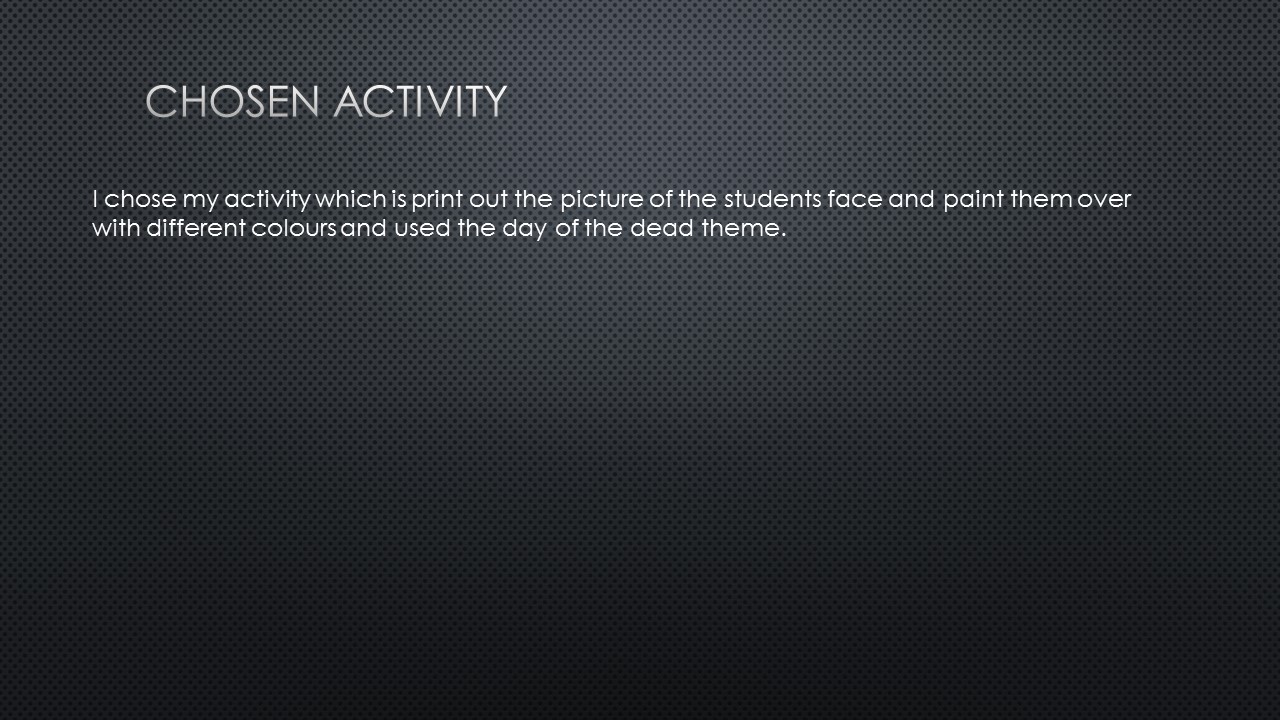The image is a rectangular screenshot of a PowerPoint slide with a grayish background adorned with small dots. The corners and edges of the slide are notably darker, while the middle section is slightly lighter, creating a subtle gradient effect. The slide contains a total of three lines of text—all in a glowing white-to-gray gradient that gives the text a slight 3D appearance. At the top, in all capitalized letters, the title reads "CHOSEN ACTIVITY." Below the heading, the two lines of text state: "I chose my activity, which is print out the picture of the student's face and paint them over with different colors and use the Day of the Dead theme." The text occupies approximately one third of the slide’s area. The overall design leads the viewer’s eye from the darker corners towards the lighter middle, guiding them naturally to focus on the text.